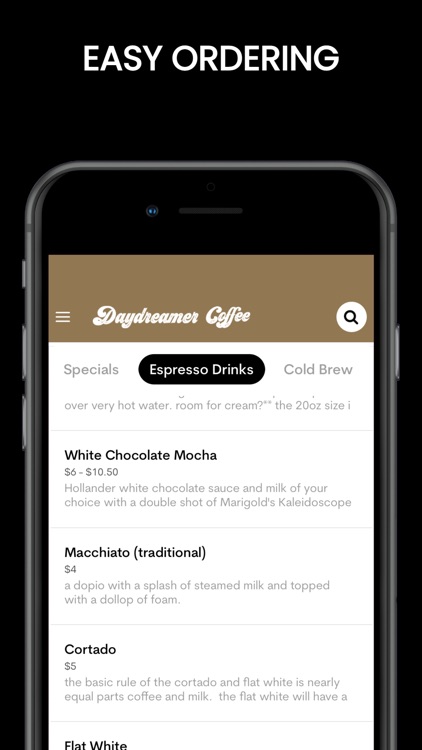A visually striking image presents a modern mobile app interface set against a sleek black background. The app, titled "Daydreamer Coffee," features a navigation bar at the top with a brown hue, showcasing the app’s name flanked by a navigation button and a search icon encased in a white circle. Beneath this header, three tabs are visible: "Specials," "Espresso Drinks," and "Cold Brew," with "Espresso Drinks" being highlighted.

Displayed prominently are drink options:
1. **White Chocolate Mocha** - Priced at $6.10, this drink includes Hollander white chocolate sauce and your choice of milk, combined with a double shot of Marigold's Kaleidoscope.
2. **Macchiato (Traditional)** - A traditional Adopio with a splash of steamed milk and topped with a dollop of foam, priced at $4.00.
3. **Cortado** - For $5.00, this drink adheres to the basic rule of nearly equal parts coffee and milk.

Unfortunately, the flat white description is partially cut off, offering only a glimpse of its preparation details. The app sports a clean, modern design style, emphasizing user-friendly navigation and clear, enticing visuals of the available coffee options.